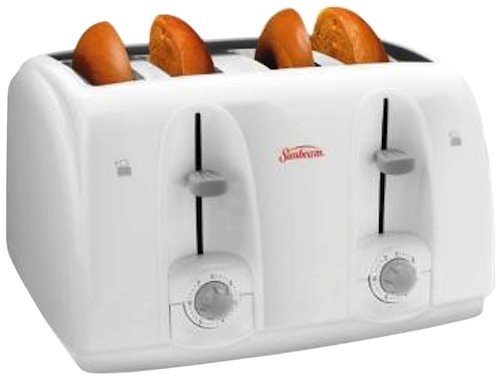This image likely from an online advertisement features a detailed close-up of a four-slot white Sunbeam toaster, each slot holding a dark brown, well-toasted bagel half. The toaster is equipped with dual independent control systems, allowing customization for each pair of slots. Each side has its own lever for lowering the toast, situated just above a gray dial marked with numbers from one to six, used to adjust the darkness level of the toast. The toaster's design is rectangular and sturdy, with the brand name "Sunbeam" prominently displayed in red lettering near the top center. The overall composition, quality of the image, and the perfectly golden and crispy appearance of the bagels make it look like a professional advertisement photo.